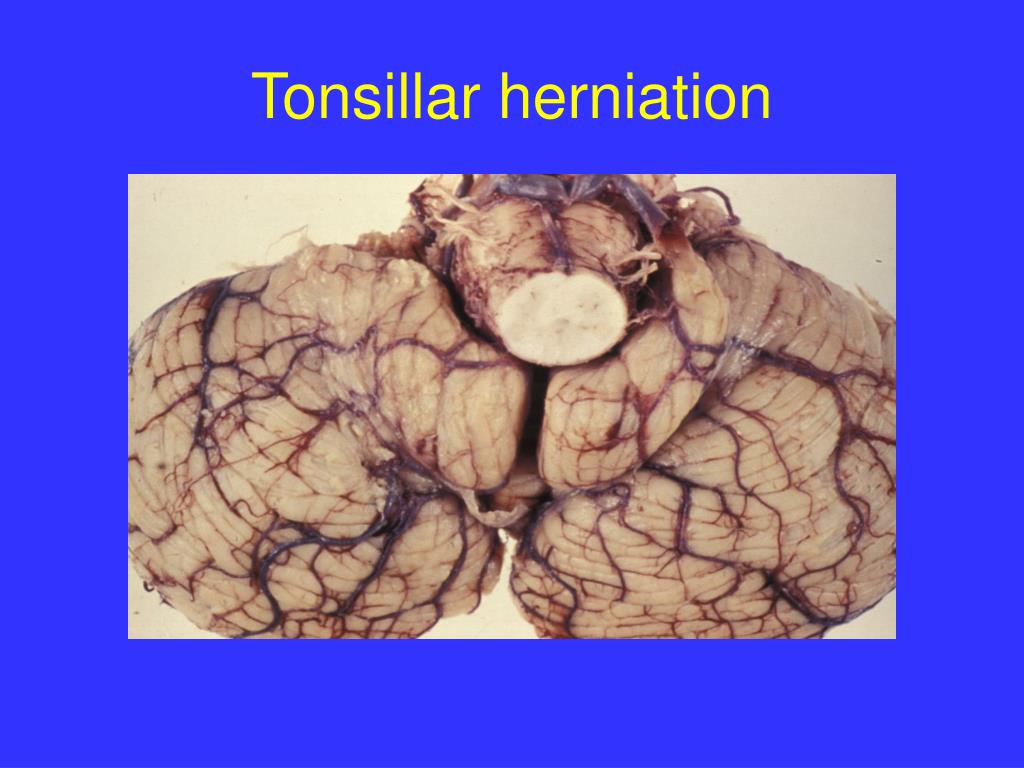The slide, titled "Tonsillar Herniation" as indicated by the yellow text at the top, features a medical image against a blue background. The central graphic is a detailed biological photo showing internal organs that seem to be mammalian, likely human. The organ depicted appears whitish with prominent red veins running throughout, alongside a white circular section near the top devoid of veins, suggesting it has been cut off. The structure includes a brownish hue with darker veins and consists of sacs on either side connected by a central tube, which seems to have been sliced. The visual arrangement suggests a focus on demonstrating the condition of tonsillar herniation.